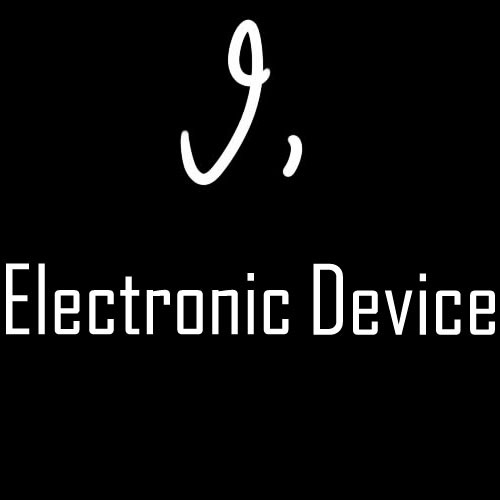The image displays a black rectangular background featuring white writing in the foreground. Dominating the top half is a prominent, curvy cursive letter, likely a capital "J" or possibly a "G," followed by a cursive comma. This cursive element is noticeably larger and distinct in style compared to the text below it. Underneath, in a more compact and blocky Courier-like font, are the words "ELECTRONIC DEVICE," with both "E" and "D" capitalized. The overall design is stark, with the contrast between the cursive and blocky fonts emphasizing the difference in style and size, set against a plain black background with no additional colors or imagery.